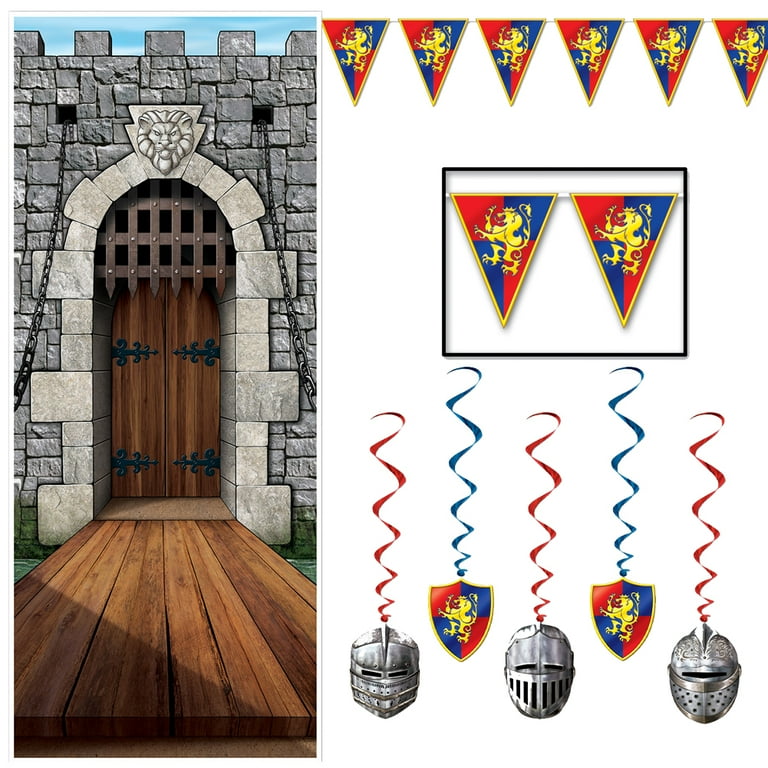The composite image features a detailed scene of a medieval castle entrance and associated heraldic designs. On the left, the castle's entryway is depicted with its gray brick walls and an arched stone archway. The closed wooden door, reinforced with black iron hardware, stands prominently, with a small drawbridge made of wooden planks extending outwards. This drawbridge is secured by metal chains that descend from the castle’s wall.

On the right side of the composite image, various medieval banners and crests are displayed. At the top, a series of red and blue triangular flags are lined up, each emblazoned with a yellow lion in the center. Below these flags, there are two rectangular close-ups showing the same flag design. Underneath, there are two shield-shaped crests bearing the same lion insignia and a set of three silver metallic warrior helmets, each adorned with either blue or red ribbons. The background of this right section is white, highlighting the vivid medieval elements. This detailed imagery suggests elements that may be utilized in a video game for designing a castle scenario.